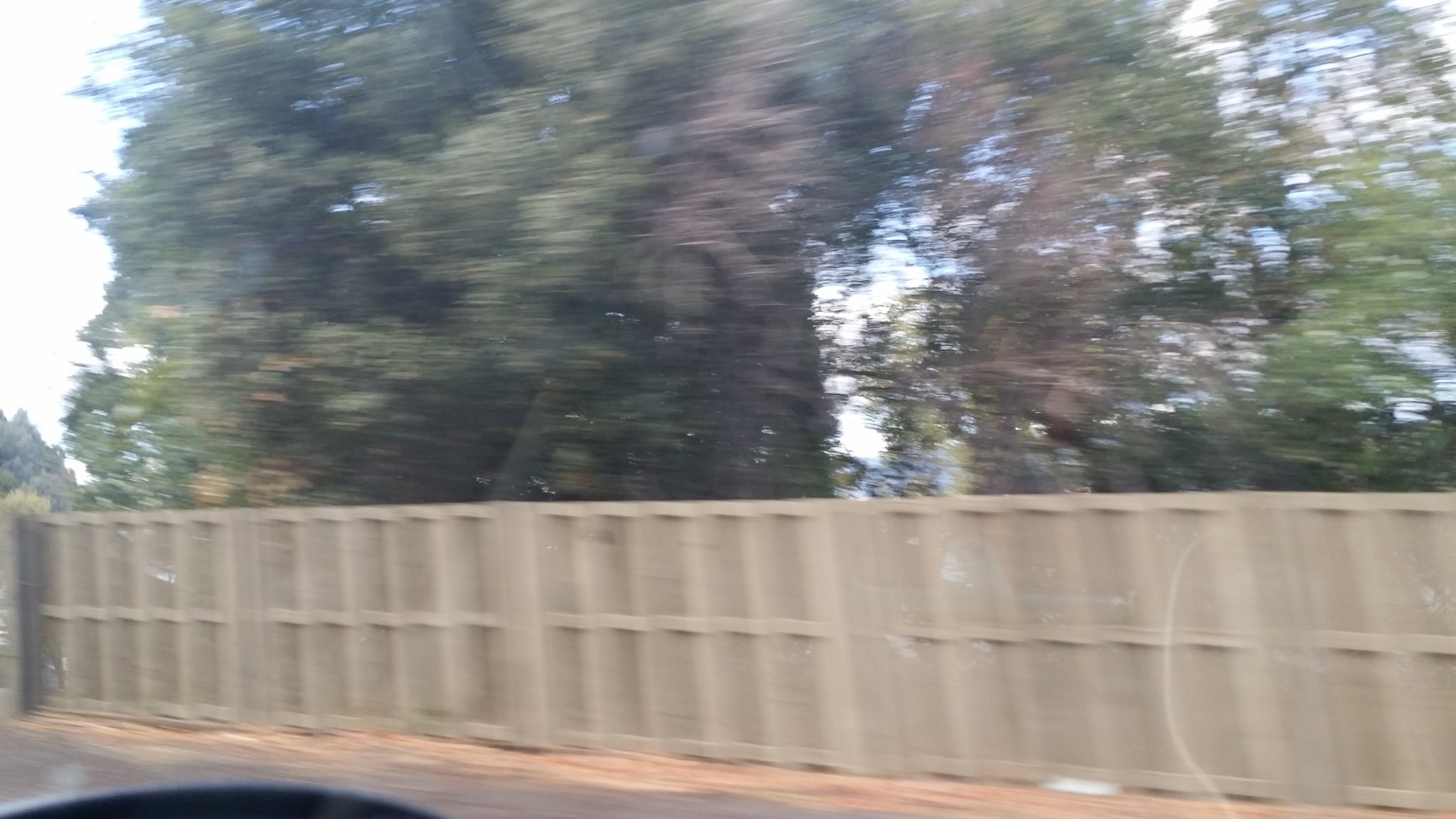This image, taken from inside a moving car, captures a landscape scene in a blurry yet detailed manner. The central focus is a brown fence, which appears to be made of concrete, situated perhaps on a bridge or alongside a road. This fence is not flat but segmented, and it stretches across the entire width of the image from the bottom left to the right-hand side. Below the fence, there's a ground cover that looks like sand or dirt, and some orange leaves are visible on the asphalt-gray road beneath. 

Behind the fence, a large, impressive tree dominates, displaying a mix of red and green foliage. The top half of the image is filled with additional trees and dense foliage, predominantly green with some brownish leaves interspersed. Small patches of the blue daytime sky peek through the upper left area. The entire scene is enveloped in a sense of motion, as evidenced by the elongated, blurry trees and the overall haze, suggesting the photo was snapped while the car was in transit.